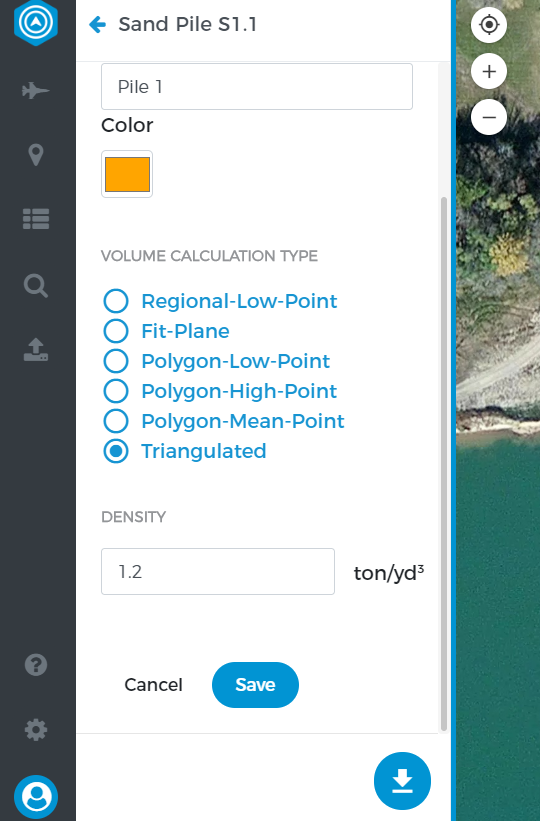In the foreground, a screen capture displays a detailed interface from a software application labeled "Sandpile S1.1." The interface shows a window with the header "Pile 1." Beneath this header, various settings and options are specified: the color is set to Orange, and the Volume Calculation Type is selected as Regional Low Point with "Triangulated" chosen among other options like Fit Plane, Polygon Low, Polygon High Point, and Polygon Mean Point. The density is entered as 1.2 tons per cubic yard (notated as ton/yd³). Two buttons, "Cancel" and "Save," are present at the bottom of the window, with "Save" highlighted as the selected option. A download icon is visible at the lower right corner of the interface.

In the background, a dark stripe on the left side of the screen contains clickable options, and to the right, the screen displays an intriguing landscape view. This image creates an optical illusion, depicting what appears to be a body of water at the bottom transitioning into gravel, then bushes, and finally grass at the top. The intriguing aspect of this image is its reversible nature; the body of water could also be interpreted as the sky, showcasing a fascinating visual ambiguity.